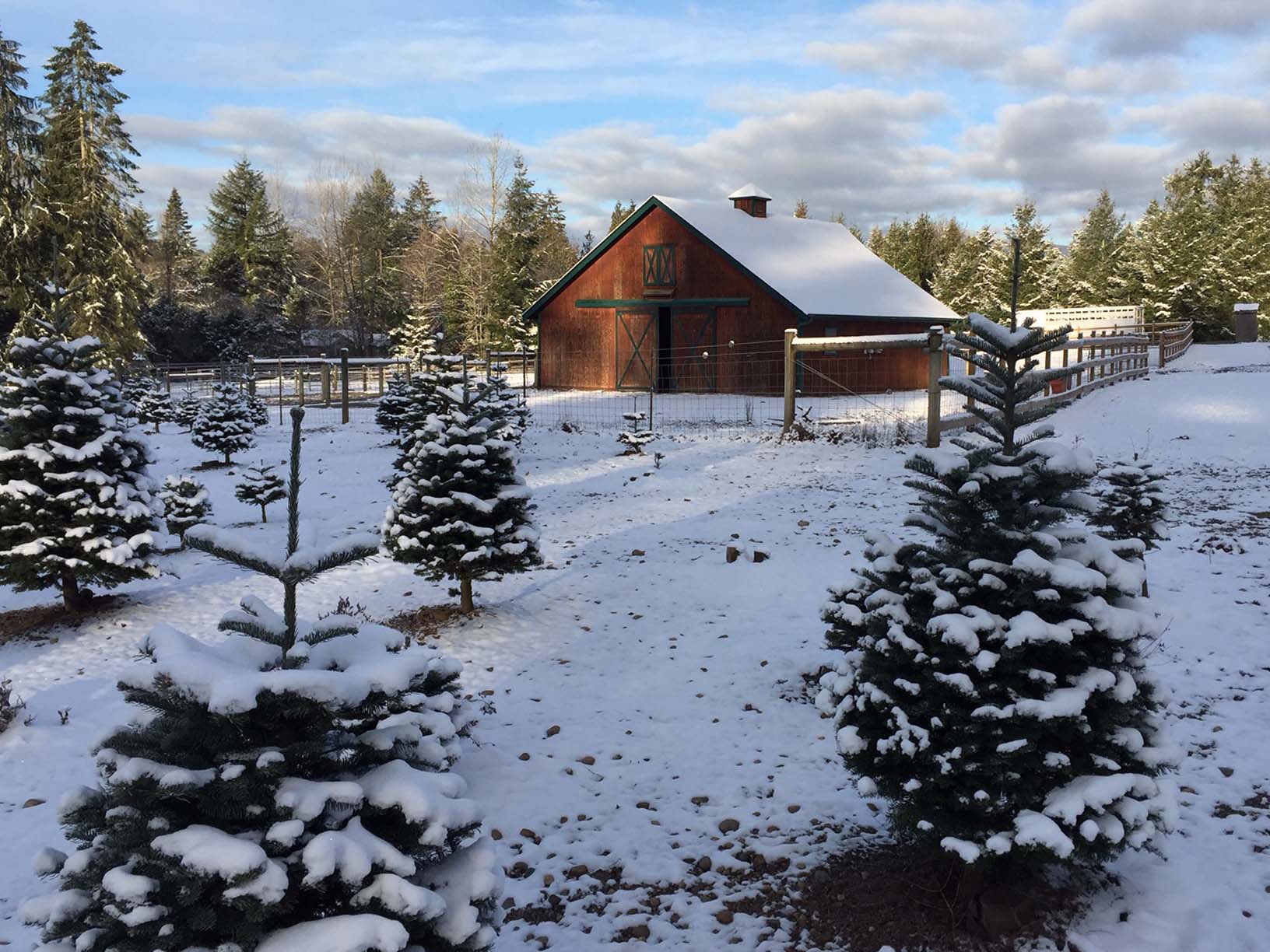In the center of this scenic daytime photograph, a large wooden barn, adorned with green trimmings and X-marked barn doors, stands majestically amidst a wintry landscape. The V-shaped, snow-covered roof is accented by a chimney, adding to the rustic charm. The barn doors, one slightly ajar, hint at the warmth inside, though the view is obstructed. A surrounding fence, transitioning from wood to wire, encloses the structure. In the foreground, small bushes resembling Christmas trees are dusted with fresh, frothy snow, while the background reveals taller evergreen trees cloaked in white, delineating the property's boundary. Above, a partly cloudy sky, tinged with blue, frames the peaceful, snow-covered scene, adding a tranquil atmosphere to the picturesque farmland.